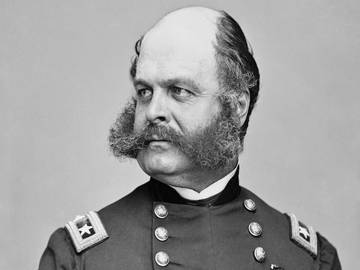This black-and-white historical photograph depicts Ambrose Burnside, a Union general from the Civil War era, who also served as the governor of Rhode Island. In the image, Burnside is attired in a dark military jacket adorned with patches on the shoulders, each featuring at least one visible star, indicating his rank. The jacket has three visible buttons on either side of the midline, and a white shirt collar is peeking out from underneath. General Burnside, a balding man with hair on the sides of his head, is most famously known for his distinctive facial hair: very large, thick mustache and sideburns that extend all the way to his ears. He is gazing to his right, off-camera, against a plain gray background.